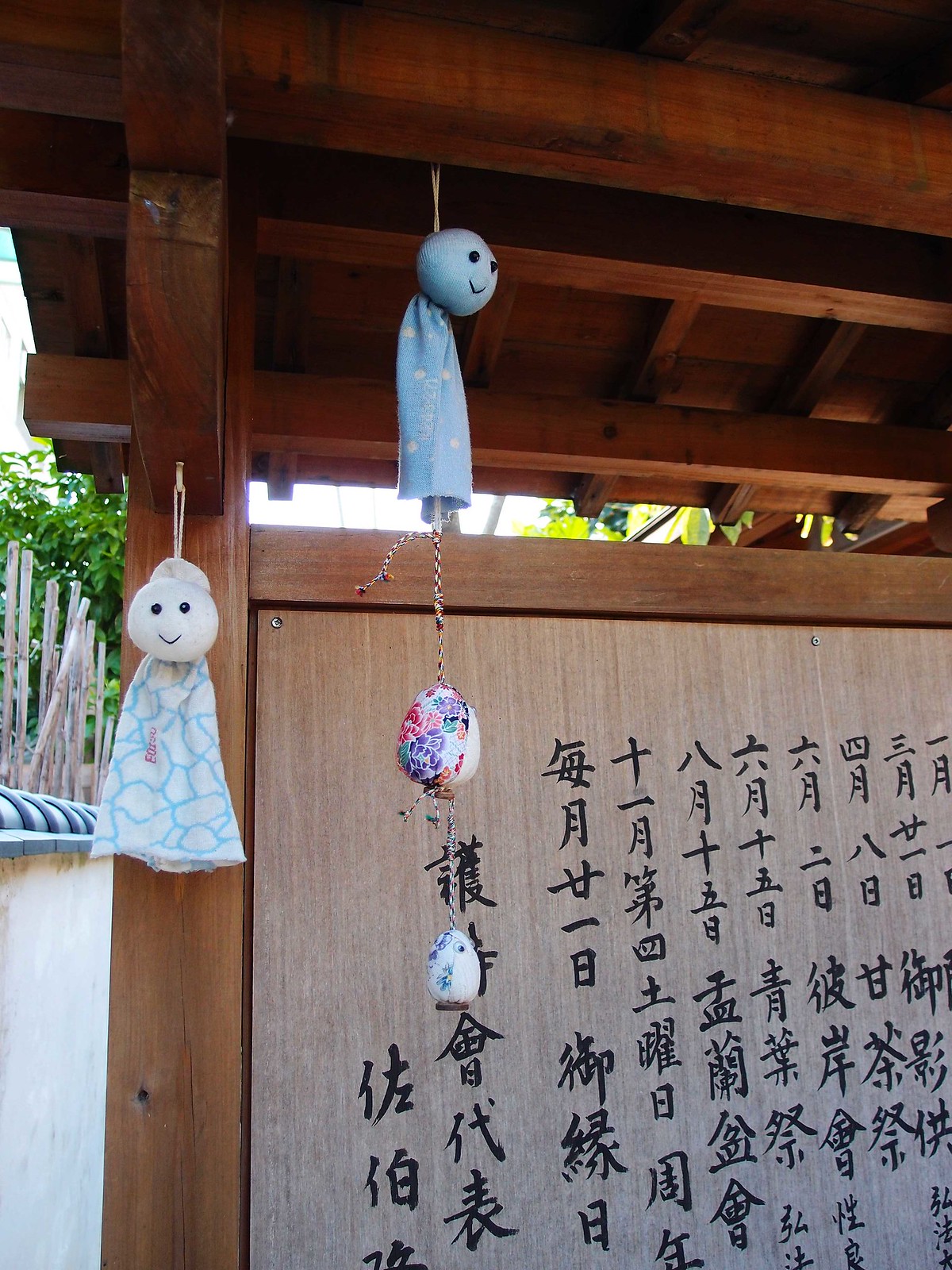In this outdoor image, likely taken in someone's backyard in the middle of the day, there is a variety of colors including tan, brown, black, purple, red, pink, green, light blue, and blue. At the top of the image, wooden rafters are visible, reminiscent of the underside of a deck. Hanging from these rafters are what appear to be two ghost-like stuffed characters. One of these characters is adorned in a dress and carries a multicolored bag. The characters are centrally positioned in the image. On the right side of the wall, Asian script is written, although it cannot be read. The left side of the image features a wall, a fence, and some bushes.